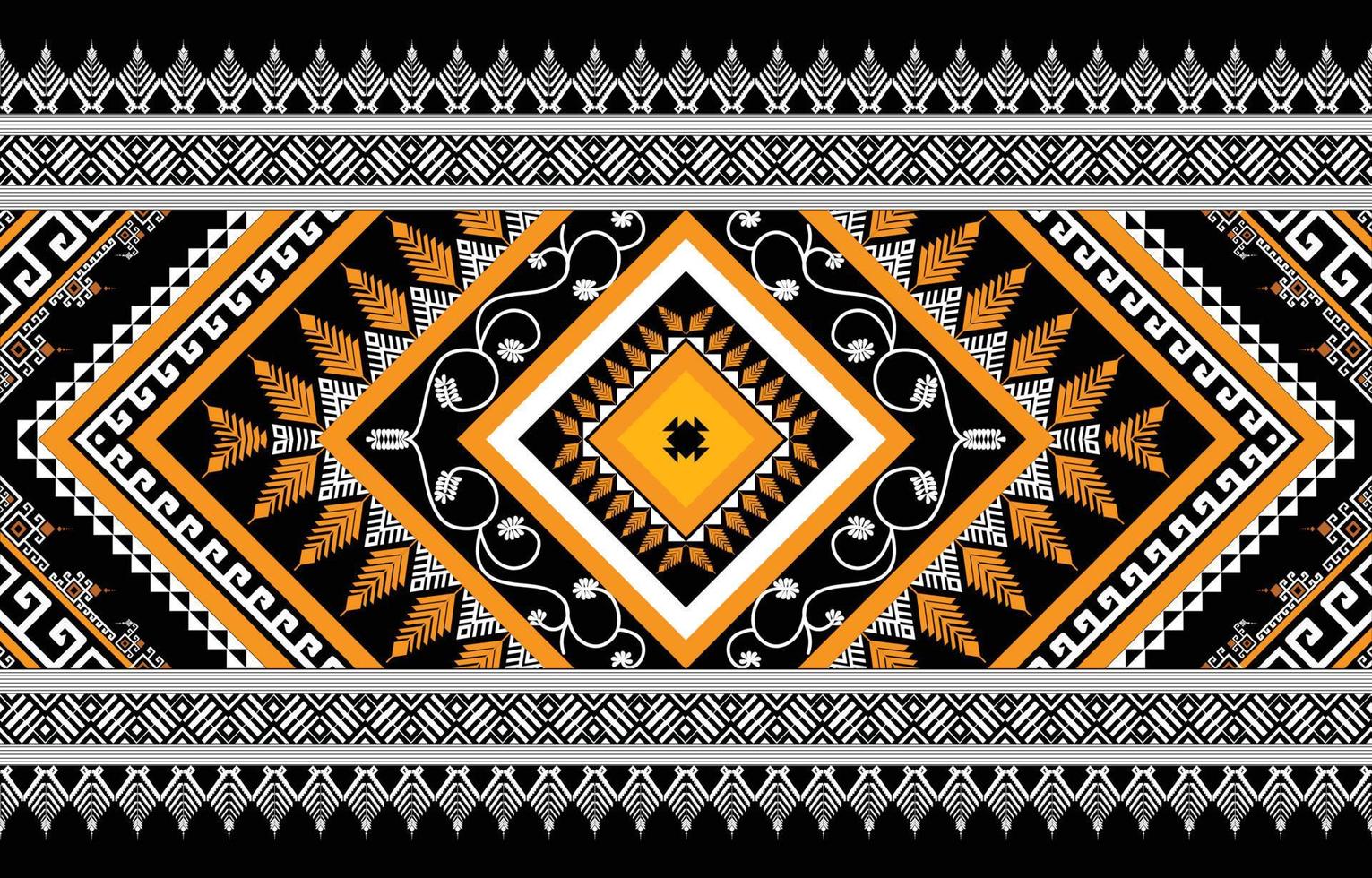The image depicts an intricate and highly detailed digital print resembling a textile, possibly inspired by Mesoamerican or Arabic designs. At the center is an orange diamond containing a black symbol composed of a smaller black diamond and black triangles. This central motif is encircled by white triangles and then orange feather-like shapes. Extending outward, the pattern continues with alternating diamonds in black, white, and orange, each containing intricate designs like plant or vine motifs. The top and bottom borders feature black backgrounds adorned with alternating white fern or fan-like shapes and stripe patterns, creating a sense of symmetry. Additional details include rows of white and black checkered and striped patterns, as well as various square motifs that expand in size towards the edges, incorporating diverse designs such as floral patterns and fern shapes. The overall color palette primarily includes black, white, and shades of orange, and the complexity of the pattern increases as it radiates outward, maintaining a cohesive yet evolving theme.